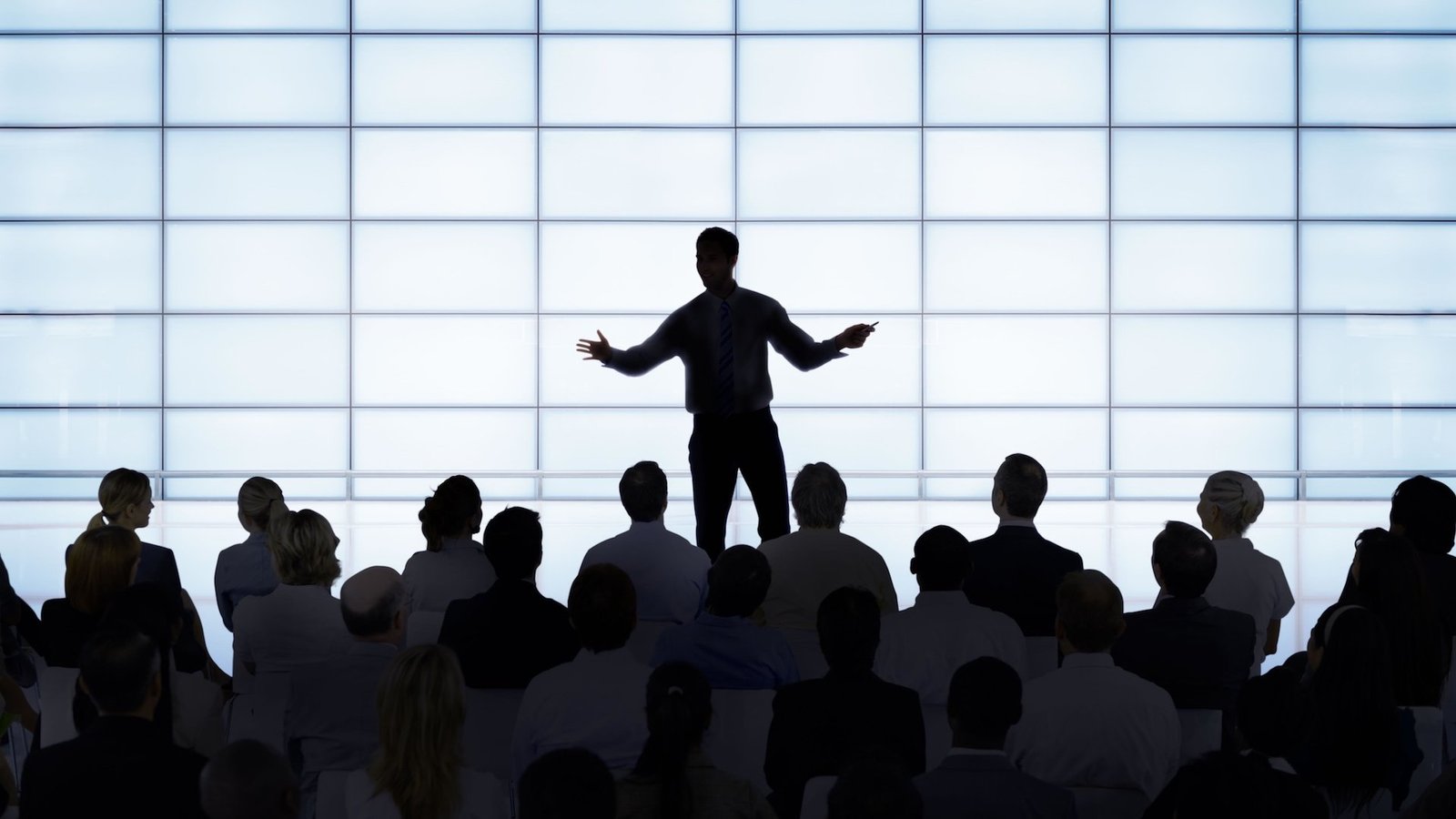In this color, landscape-oriented photograph, a man is giving a dynamic presentation on a sleek, glossy white stage in front of a captivated audience. Both the speaker and the audience are rendered in silhouette, creating a striking contrast against the brightly illuminated backdrop. The back wall of the stage features a grid of horizontally aligned, glowing rectangular panels separated by gray lines. The speaker, positioned centrally with his head turned slightly to the left, exudes charisma. His left arm is outstretched with open fingers, and his right hand, almost level with his chest, holds a sharp object, possibly a pointer. Below the stage, the darkly lit crowd includes visible details such as a woman with a ponytail on the far right, her nose tip visible as she faces the speaker. The entire audience is intently focused on the presenter, enhancing the compelling atmosphere of this business or formal event.